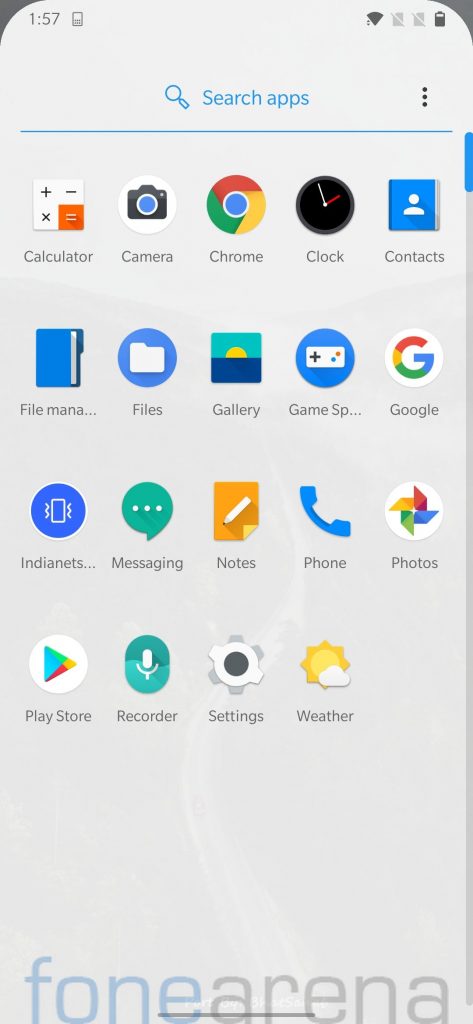The displayed image is a screenshot from a smartphone showing its "Search Apps" page. At the top of the screen, the time is displayed as 1:57, located in the left-hand corner. The status bar reveals a nearly full battery icon, indicative of the device being an iPhone. Below the status bar, there is a search bar allowing users to type and search for different applications.

The main section of the screenshot showcases various app icons arranged neatly across the screen. These icons include: 
- Calculator
- Camera
- Chrome
- Clock
- Contacts
- File Manager
- Files
- Gallery
- Game app
- Google
- Messaging
- Notes
- Phone
- Photos
- Play Store
- Recorder
- Settings
- Weather

Prominently displayed at the bottom of the screen, in large text, is the title "FONEARENA."

The overall screenshot presents a clear and organized layout of available applications on the smartphone, providing a comprehensive view of the apps and features accessible to the user.